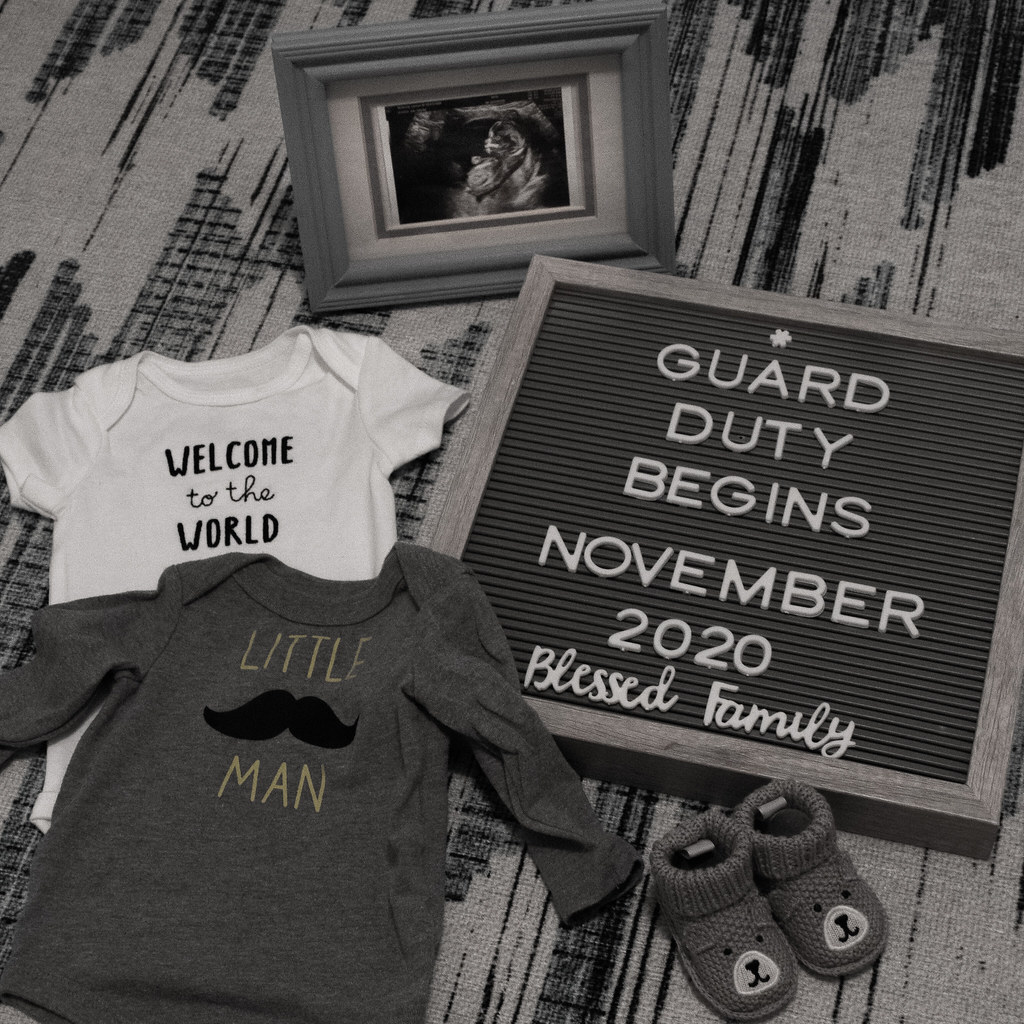This black and white image appears to be a detailed baby announcement arranged on a patterned material. In the background, there's a framed ultrasound picture of a baby, possibly set on a bed. On the left side of the image, there are baby clothes including a white onesie that says "Welcome to the World" and a gray shirt with the phrase "Little Man" separated by a black mustache. Towards the right, there is a picture frame displaying the text "Guard Duty Begins November 2020, Blessed Family." Closest to the front of the image are small teddy bear booties.